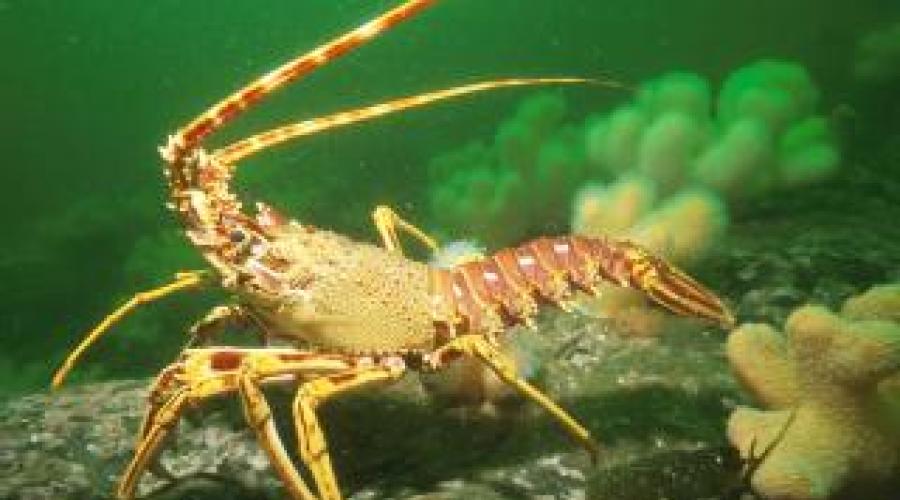The image depicts an underwater scene bathed in a murky greenish tint. Dominating the center is a creature resembling a hybrid of a lobster and a crab, displaying a mottled shell of deep reddish-brown and yellowish sand tones. The creature possesses numerous long legs and tentacles, with prominent yellowish crab-like claws. Its tail, similar to a lobster's, extends to the right, while its head is oriented to the left, with two long antennas protruding from its raised head and pointing backward. The bottom right corner of the image features a tan coral structure, and a stony formation with white spots resides further to the left, adding texture to the underwater terrain. The animal appears illuminated by a light source, creating a highlight on its body amidst the green, murky water that dominates the background. Overall, the scene is somewhat unclear and blurry, giving it an ethereal, otherworldly quality.